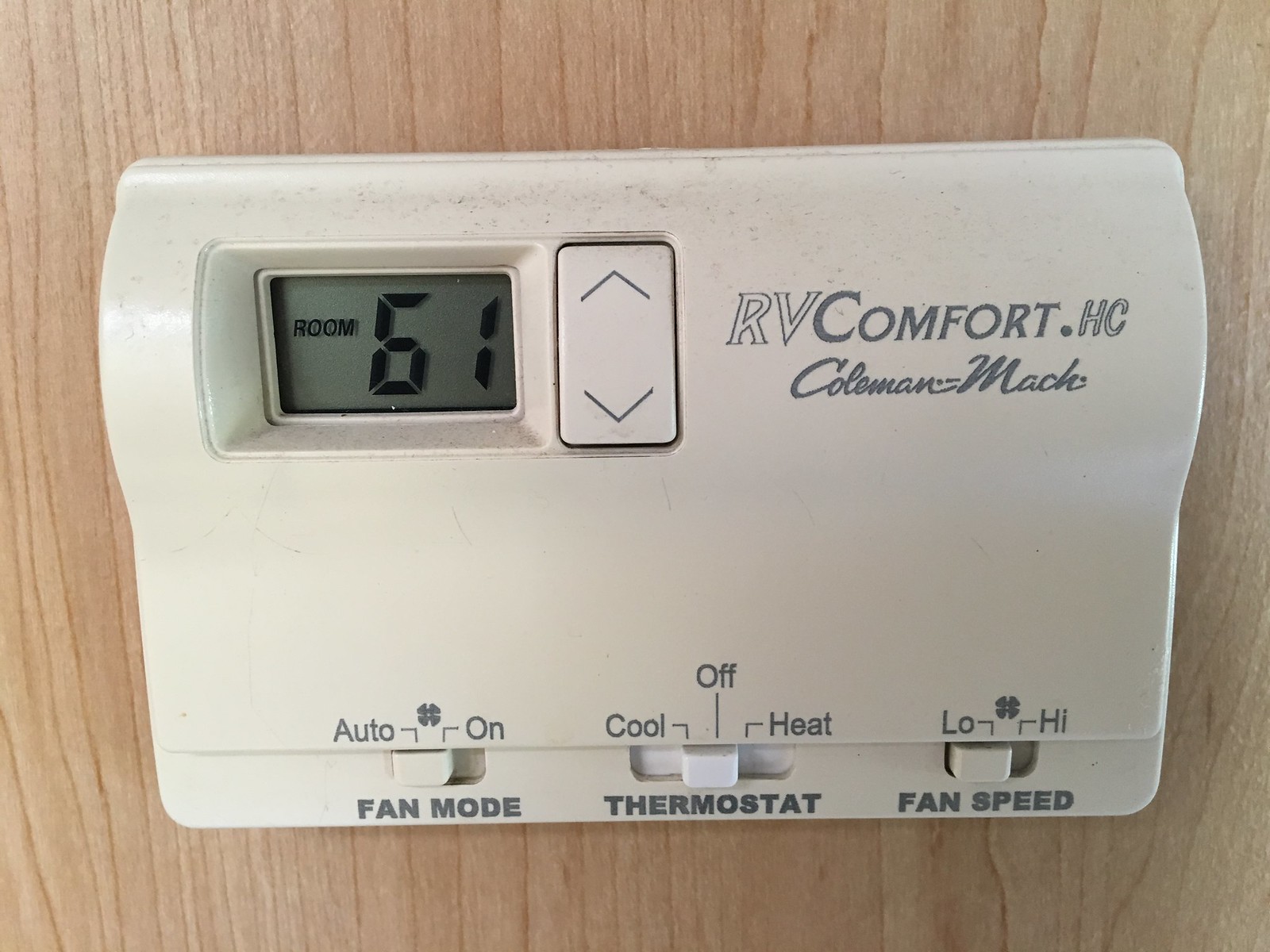The image showcases a thermostat mounted on a light wooden-colored wall. The top right corner of the thermostat features a logo that reads "RVcomfort.hc" and a cursive inscription "Coleman Match." On the small digital screen located on the left side of the device, the display reads "room 61." Adjacent to this display is a rectangular button with up and down arrows designed for adjusting the temperature settings. At the bottom of the thermostat, there are three switches. The left switch, labeled "Fan Mode," has options of "Auto" and "On," currently set to "Auto." The middle switch, labeled "Thermostat," allows for "Cool," "Off," and "Heat" settings, and is currently switched to "Off." The right switch, labeled "Fan Speed," offers "Low" and "High" settings, with the current setting on "Low."